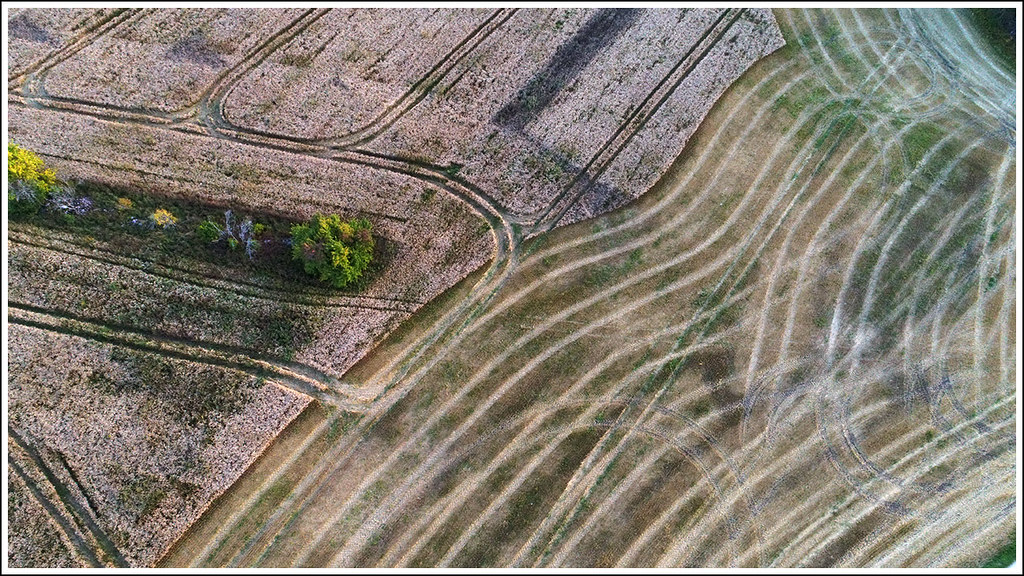The aerial photograph reveals a patchwork of meticulously organized fields interspersed with various plants, showcasing a rich tapestry of agricultural activity. The entire right-hand corner is a well-trimmed field marked by a network of tire tracks, which have left gray and brown streaks where vegetation has been crushed or compacted. Vertically intersecting tracks further influence the layout, suggesting regular vehicular movement such as tractors. On the left side, orderly rows of plants are visible, with tire marks carving out small islands of preserved plant life. In the center-left, a rectangular patch of brown soil hosts several large trees, standing out as a distinct area amid the cultivated land. The overall landscape features hues of green, brown, and yellow, reflecting varying levels of plant health and growth. The ground appears dry but arable, with indications of past or ongoing agricultural use, including what could be rows of sunflowers and other shrubs. This tapestry of fields, tire tracks, and vegetation paints a detailed picture of human interaction with the land.